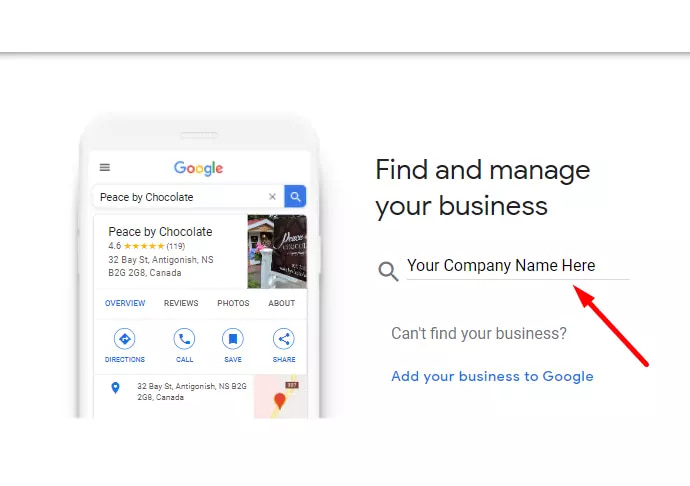The rectangular, horizontally oriented image features a main background of entirely white. At the top edge of the image, a gray border extends the full width. Below this border sits the focal point: a smartphone with a white case, displaying a Google search result for "Piece by Chocolate."

On the phone screen, the Google search bar is highlighted with the query "Piece by Chocolate" and accompanied by the blue search button with a magnifying glass icon. Directly underneath, the search result shows "Piece by Chocolate" with an impressive rating of 4.6 out of 5 stars based on 119 reviews. The information continues, noting the business's category as a pastry shop located in Antigonish, NS, Canada, and displays a small image of the shop.

Further down, the screen lists various navigation options: "Overview," "Reviews," "Photos," "About," along with buttons for "Directions," "Call," "Save," and "Share." A miniature map indicates the business's location.

On the right-hand side of the phone screen, there's a prompt reading "Find and Manage Your Business," accompanied by a red arrow pointing to "your company name here." Below this, an invitation states, "Can't find your business? Add your business to Google."

This detailed caption gives viewers a comprehensive understanding of the image, ensuring they grasp the various elements displayed on the smartphone screen within the white-bordered background.